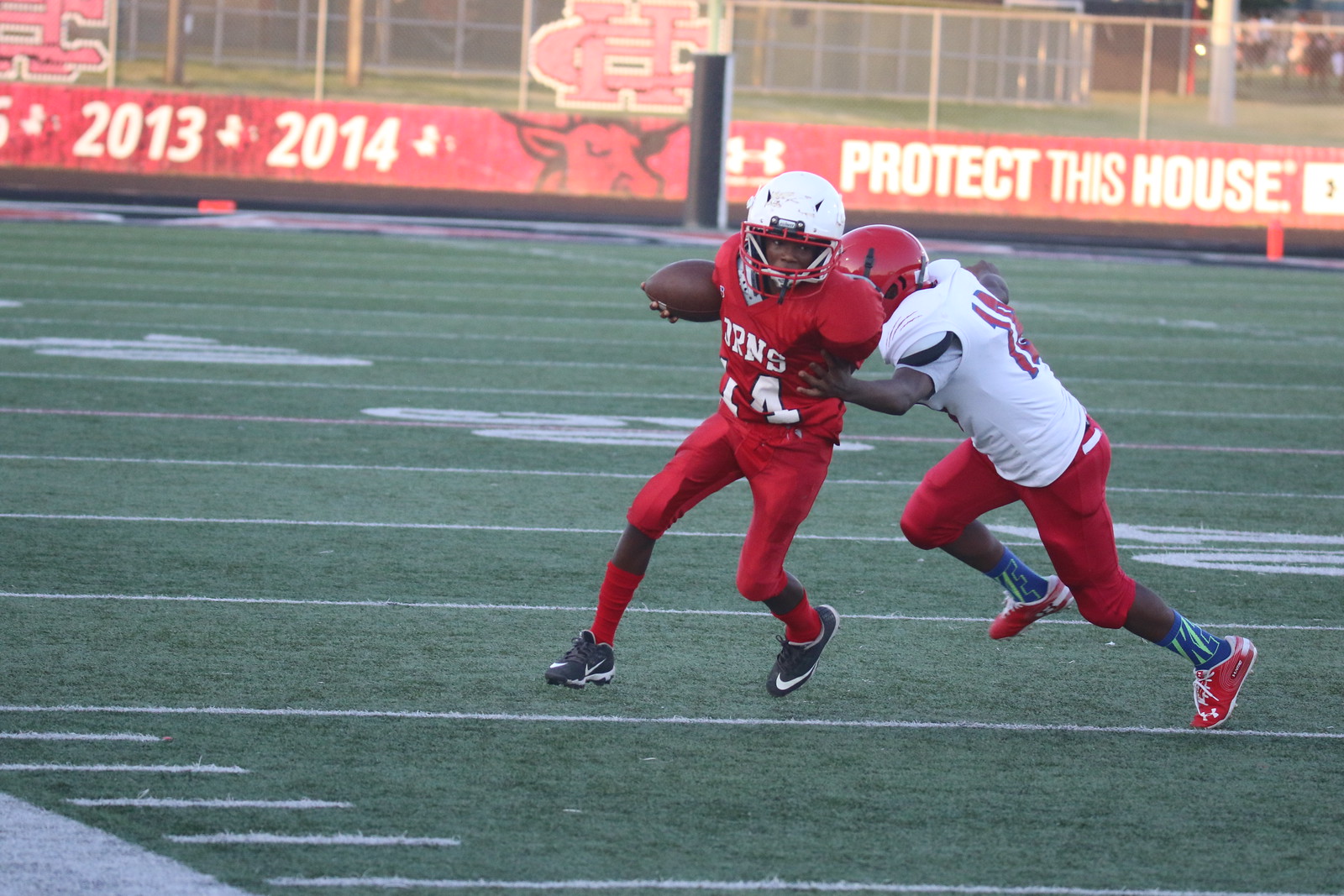In the image, two teenage black boys are intensely playing football on a turf field. The player on the left, dressed in a fully red jersey and white helmet, holds the football tightly. His opponent, in a white jersey with red lettering, red pants, and a red helmet, is in the midst of attempting a tackle. His left hand firmly grips the side of the player in red, while his right arm is outstretched, poised to pull him down. The background features a 2013-2014 season banner and an Under Armour sign with the phrase "Protect This House." The boys' contrasting jerseys highlight the dynamic action between offense and defense.